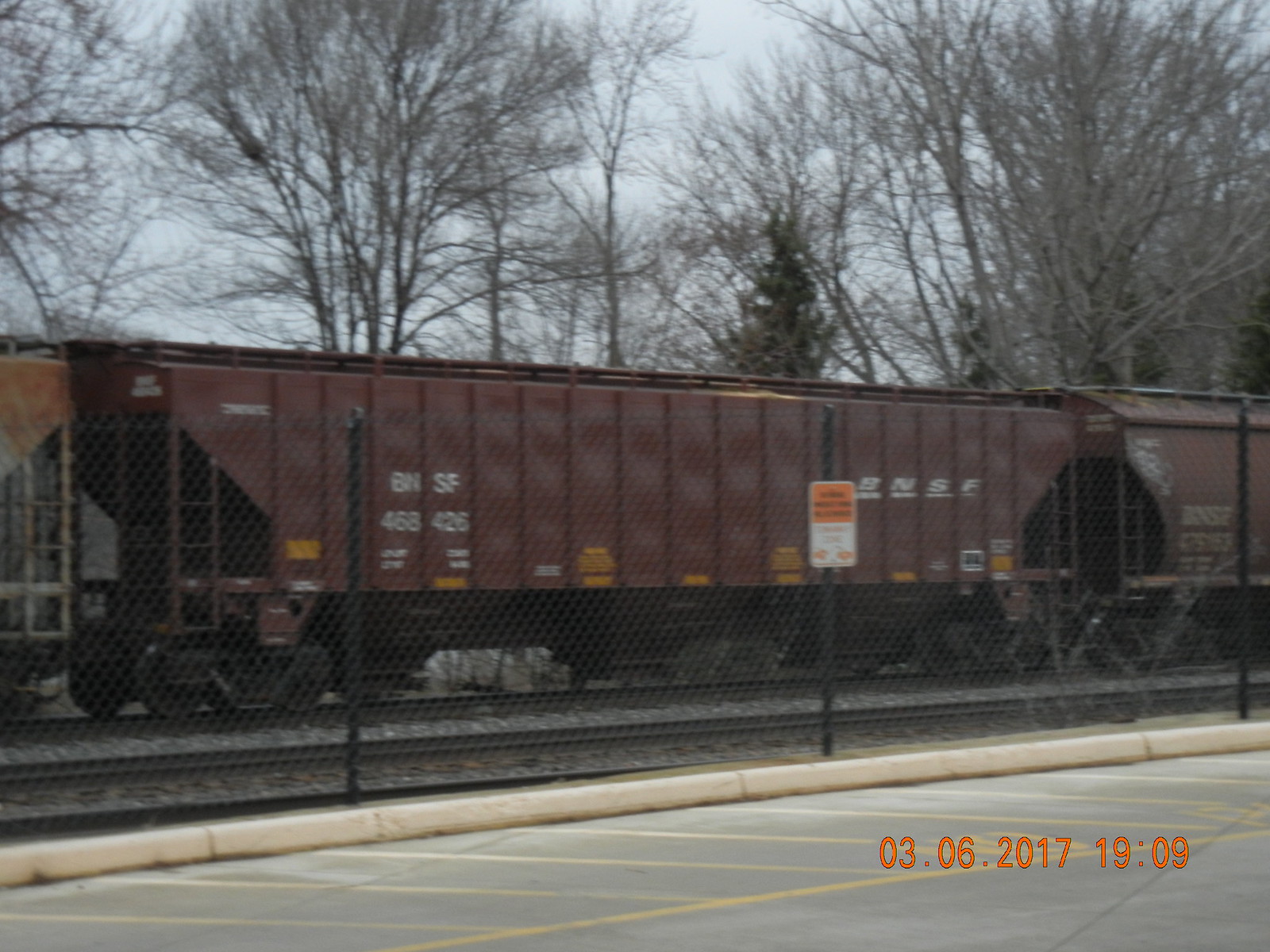This image captures a brown train car, marked with "BNSF 468426" in white lettering, moving along the tracks. The photo appears to be taken during the fall or winter, as most trees in the background are bare, except for a single pine tree retaining its needles. The sky is clear and blue, providing a crisp backdrop. In the foreground, there is a parking lot with marked spaces and a cream-colored sidewalk with a railing. Yellow lines on the road near the sidewalk suggest no parking zones. A black fence separates the parking area from the train tracks. An orange and white sign with black writing stands on a metal pole near the tracks. The bottom right corner of the image timestamps the moment as March 6, 2017, at 19:09.